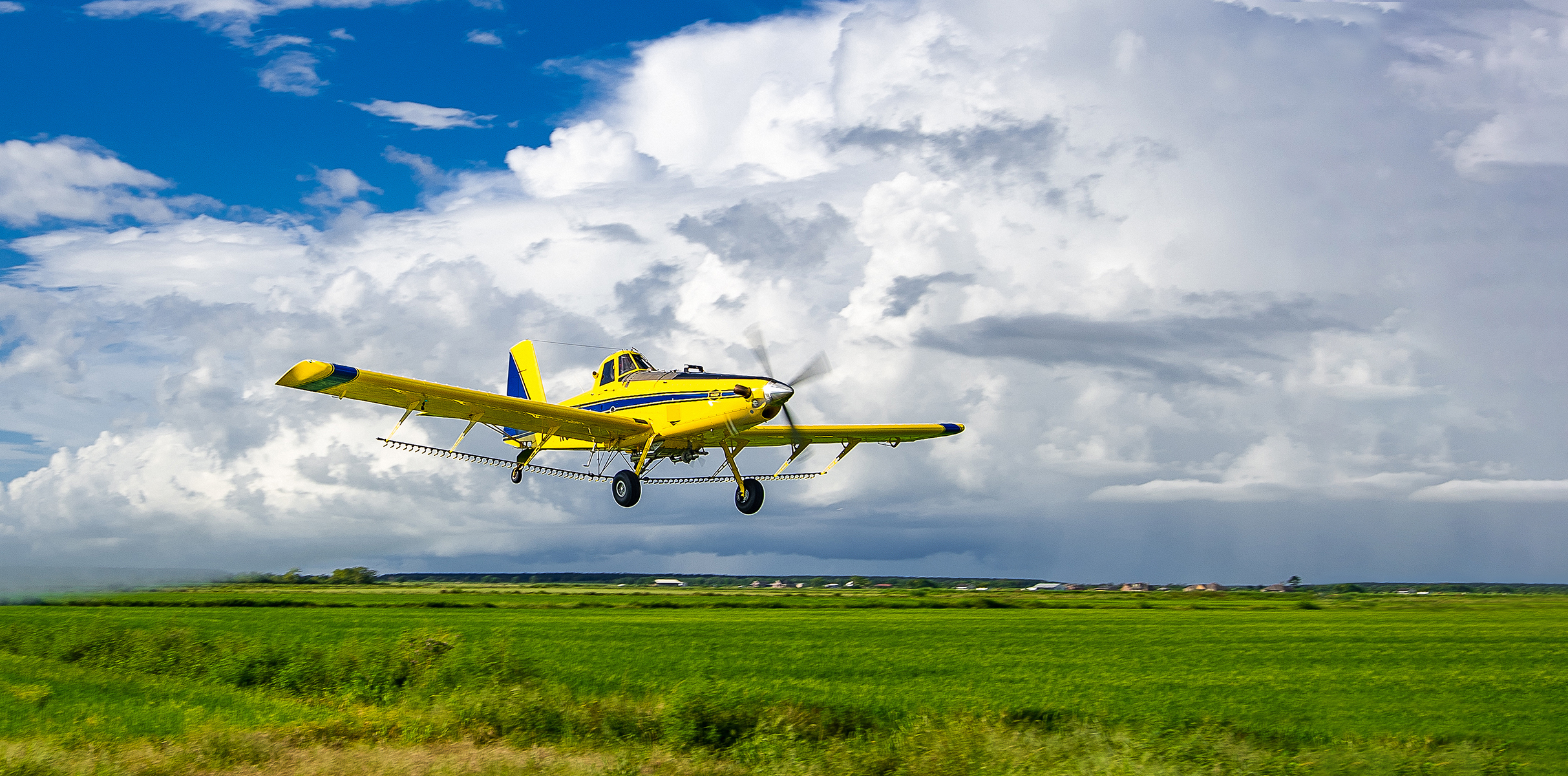The image captures a crisp, detailed scene of a small yellow propeller plane, adorned with distinctive blue stripes on its body and wings, either preparing to land or having just taken off. The black wheels, including one towards the tail, are prominently down, indicating an impending landing. The plane hovers about 20 to 30 feet above an expansive, lush green grass field, poised for a smooth descent. The backdrop features faint silhouettes of distant buildings or farm structures, adding depth to the rural setting. The sky is a mix of medium bright blue with patches of white and gray clouds, suggesting either an upcoming rain or a beautifully varied day. The vivid colors and sharp detail of the photograph highlight a single seat in the cockpit, making it clear this is a one-person aircraft.